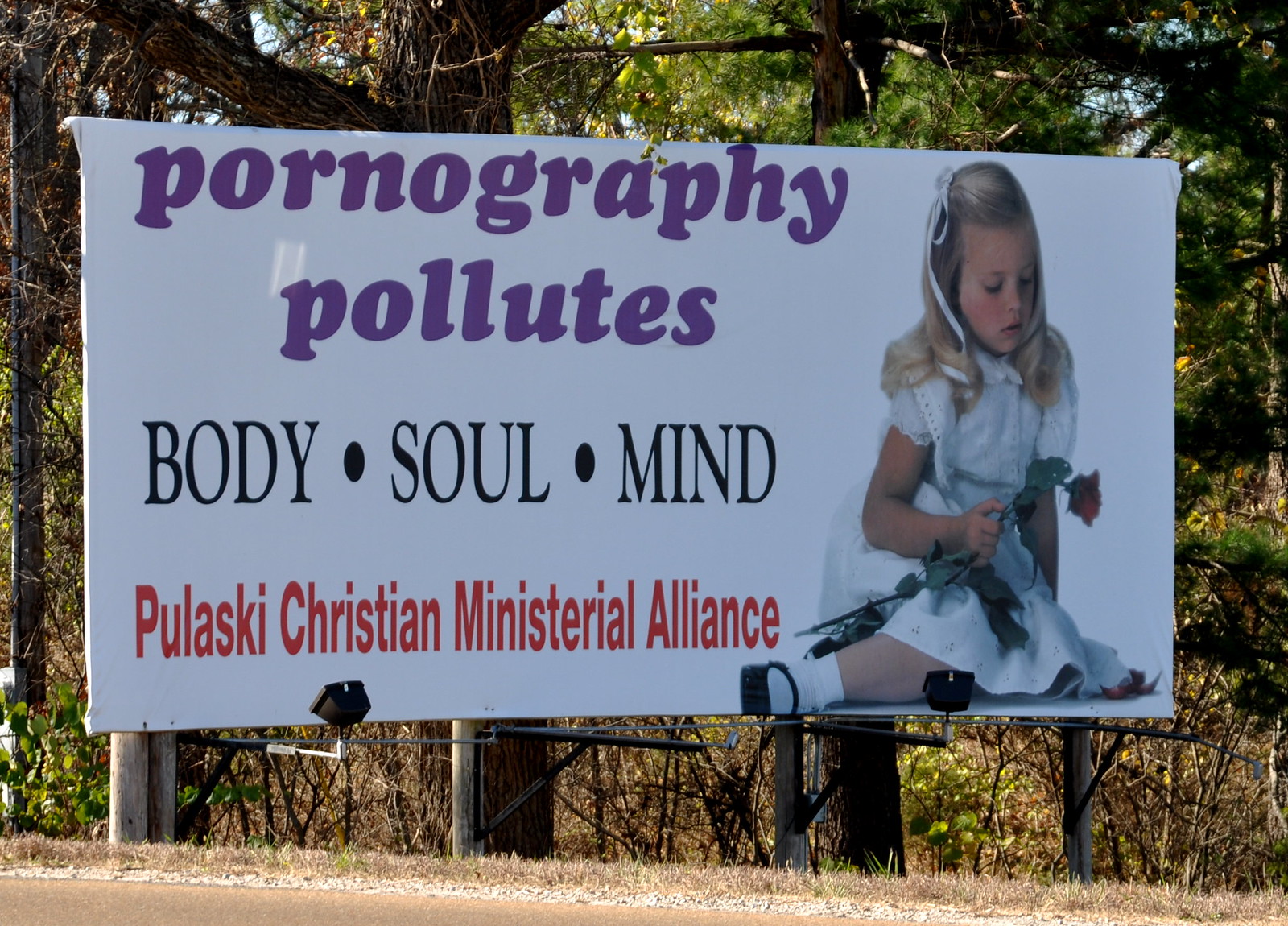The photograph features a prominent billboard set against a white background, supported by four wooden or metal posts. Four black lights are affixed to these posts and are angled to illuminate the billboard during nighttime. Positioned beside a road, the scene behind the billboard includes a serene forest with a mix of green leaves and pine needles, interspersed with the brown trunks of distant trees. The roadside is visible in the bottom left corner of the image, accompanied by a patch of brown grass beneath the billboard.

The billboard itself showcases an image of a young girl holding a rose, dressed in a pristine white dress. The text on the billboard is rendered in a combination of purple, red, and black letters, adding a burst of color against the white background. The setting, with its blend of natural elements and the striking visual of the billboard, creates a captivating scene.